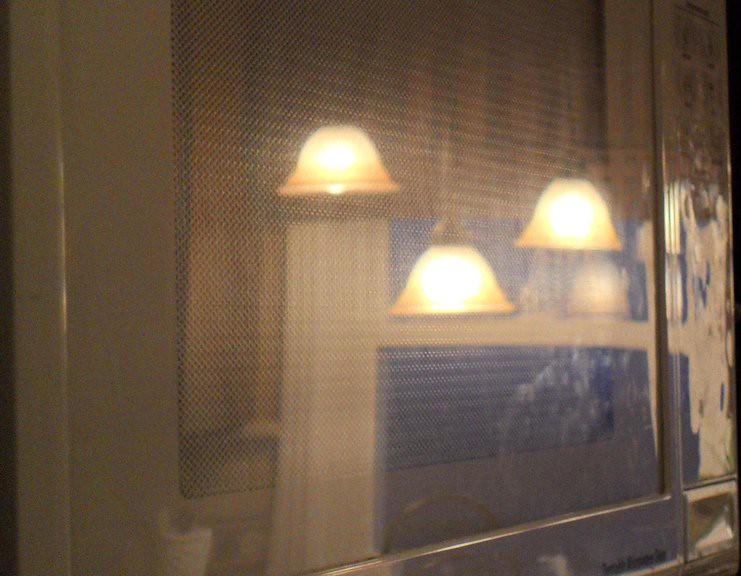This image appears to be a blurry, out-of-focus photograph taken indoors, possibly in a smoky room. The main focus is a reflection, possibly on a glass or plastic surface, such as a window or microwave door, featuring three pendant lights hanging from the ceiling. These lights emit a soft glow and dominate the center of the image. The surrounding area in the picture is difficult to discern, with only vague outlines of a white-framed window or door visible. Additionally, some faint writing is present in the bottom corners of the image, but it is indecipherable. The overall tone of the photograph is dull and lacks color, making it challenging to clearly identify other objects or details within the scene.